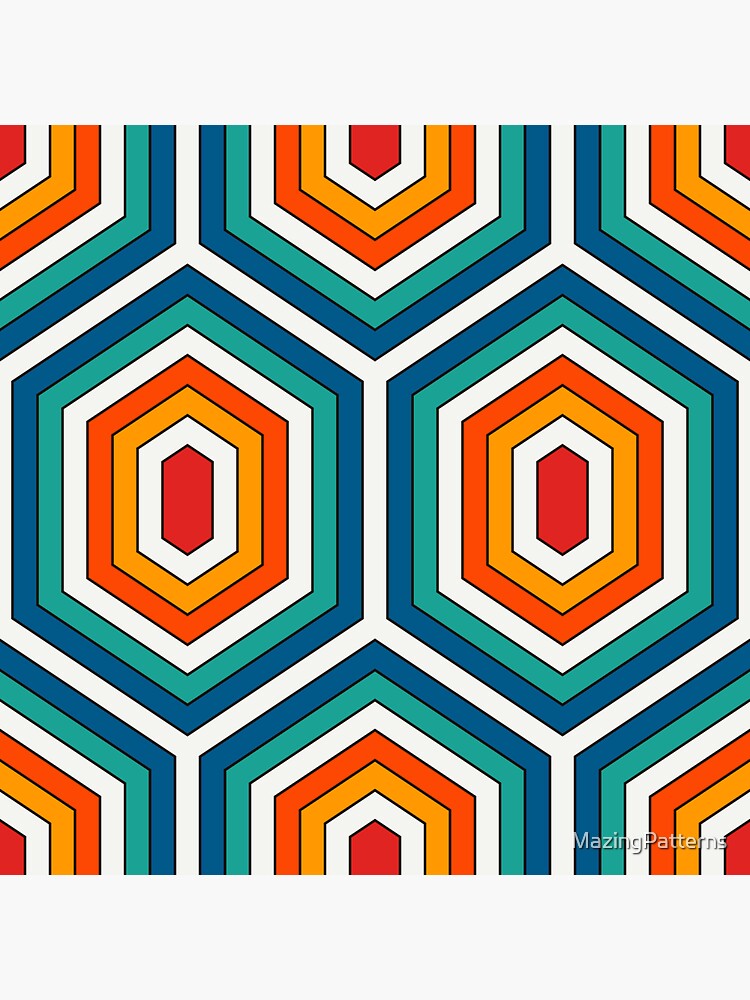The image is a highly detailed, computer-generated drawing showcasing an intricate geometric pattern designed for decorative purposes, possibly as a wallpaper. The pattern consists of a series of nested diamonds, each varying in size and color. At the center is a small red diamond, enveloped by increasingly larger diamonds in the following color sequence: red, white, light orange, bright orange, white, aqua, and finally, a dark blue diamond as the outermost layer. The design exudes a vibrant mix of colors, including blue, teal, gold, yellow, and white, structured in precise straight lines forming elongated hexagonal shapes. The entire pattern repeats itself harmoniously within a square format, and in the bottom right corner, the words "Amazing Patterns" are inscribed, further emphasizing the artistic and decorative intent of the image.